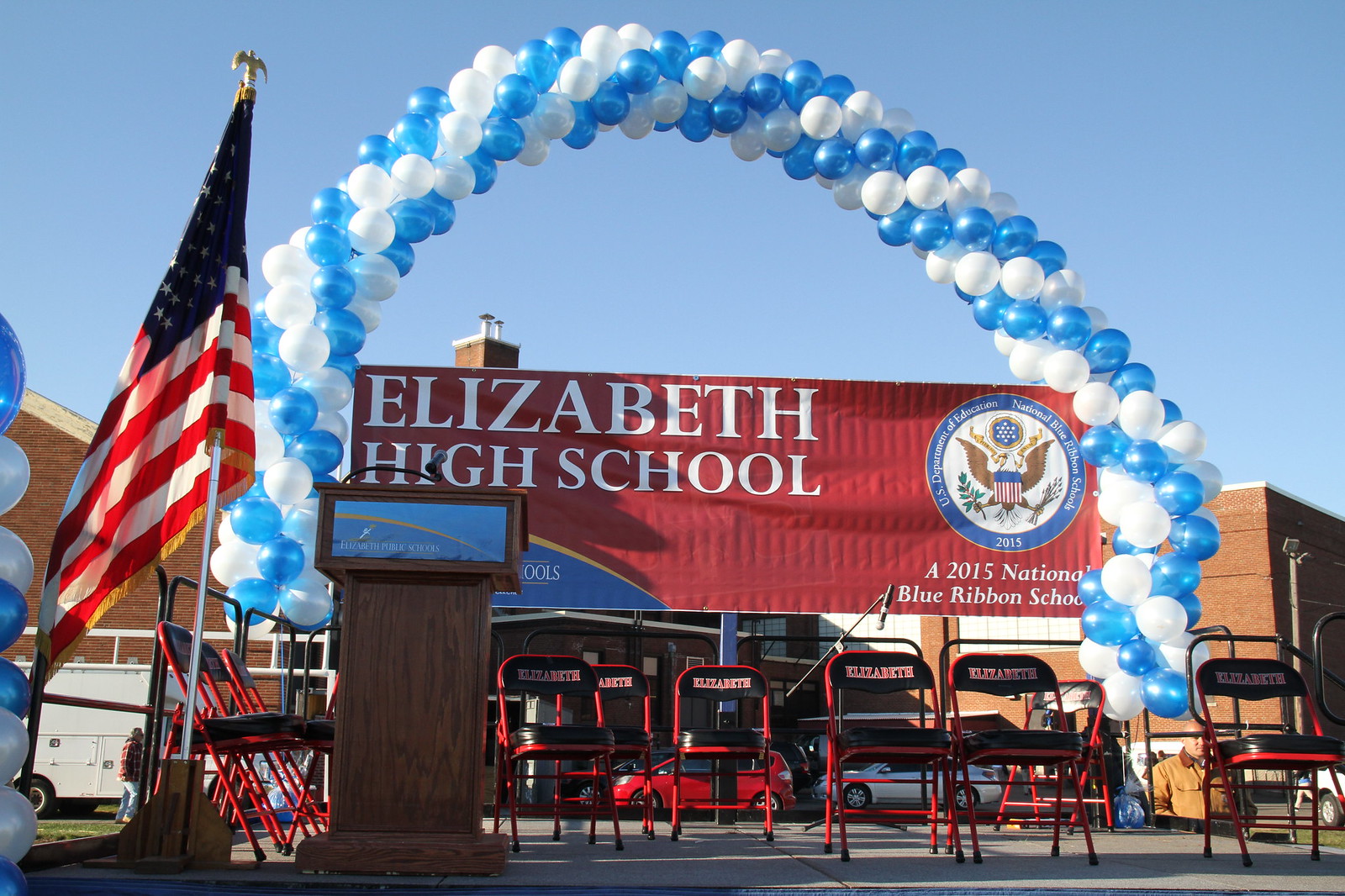This image captures a vibrant and meticulously arranged graduation scene at Elizabeth High School, prominently a 2015 National Blue Ribbon School, likely the one known in New Jersey. The focal point is a wooden podium, topped with a glass surface, positioned center-stage and accompanied by an American flag to its side. Behind the podium are numerous red chairs, suggesting an audience or participants for the event, and a festive assortment of blue and white balloons creating a decorative semi-circle arch above.

The backdrop includes the school's grand entrance with a banner that boldly reads "Elizabeth High School" in white letters against a red background. Behind this signage is a substantial brick building, stretching into the background on both left and right, notable for its small roofed entrance area. The school's logo, featuring an eagle set within a blue-bordered circle, is also visible on the banner with the year 2015 prominently displayed below it. 

In the foreground, to the left, a white truck, possibly an emergency vehicle, is parked. Additionally, various cars, such as red and gray ones, are stationed directly in front of the school entrance, enhancing the scene's bustling atmosphere of a significant celebratory event, likely a graduation ceremony.